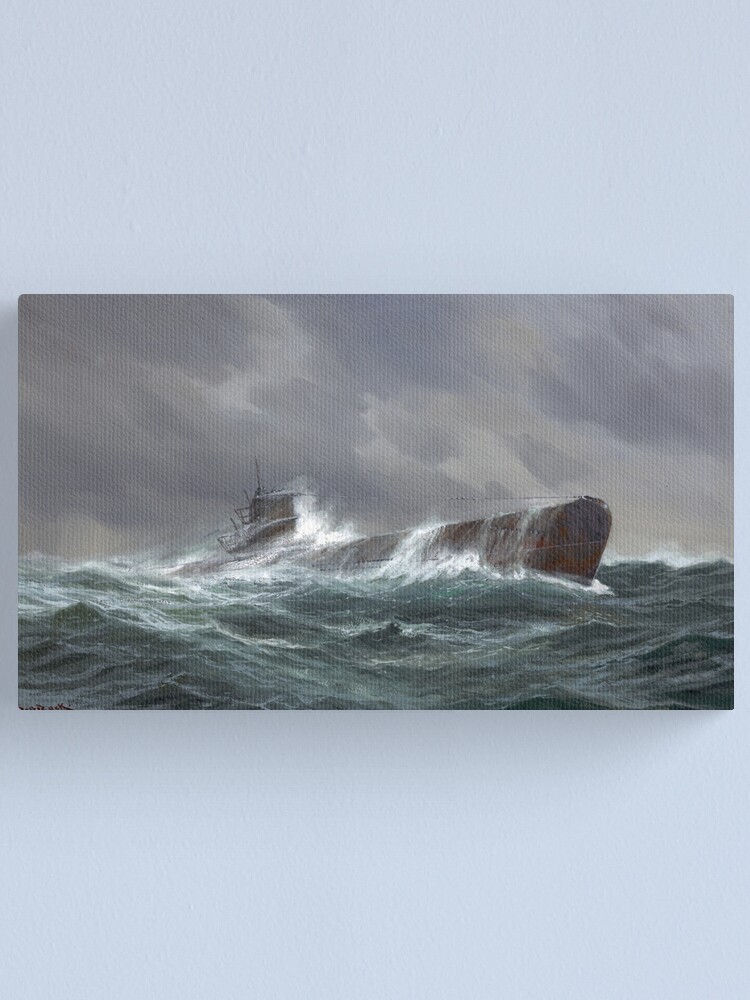The image depicts a detailed painting of a military submarine surfacing in a tumultuous ocean. The painting is rectangular, in landscape mode, and hangs unframed on a baby blue wall, casting a shadow. The submarine, with its conning tower visible, appears metallic with brown highlights and some rust, emphasizing its rugged appearance. It battles through heavy waves and stormy waters, with white spray erupting from its emergence. The sky above is a stormy gray, filled with clouds, suggesting harsh weather conditions. The vivid depiction of rough seas and the dramatic surfacing of the submarine captures the scene's intensity and foreboding atmosphere.